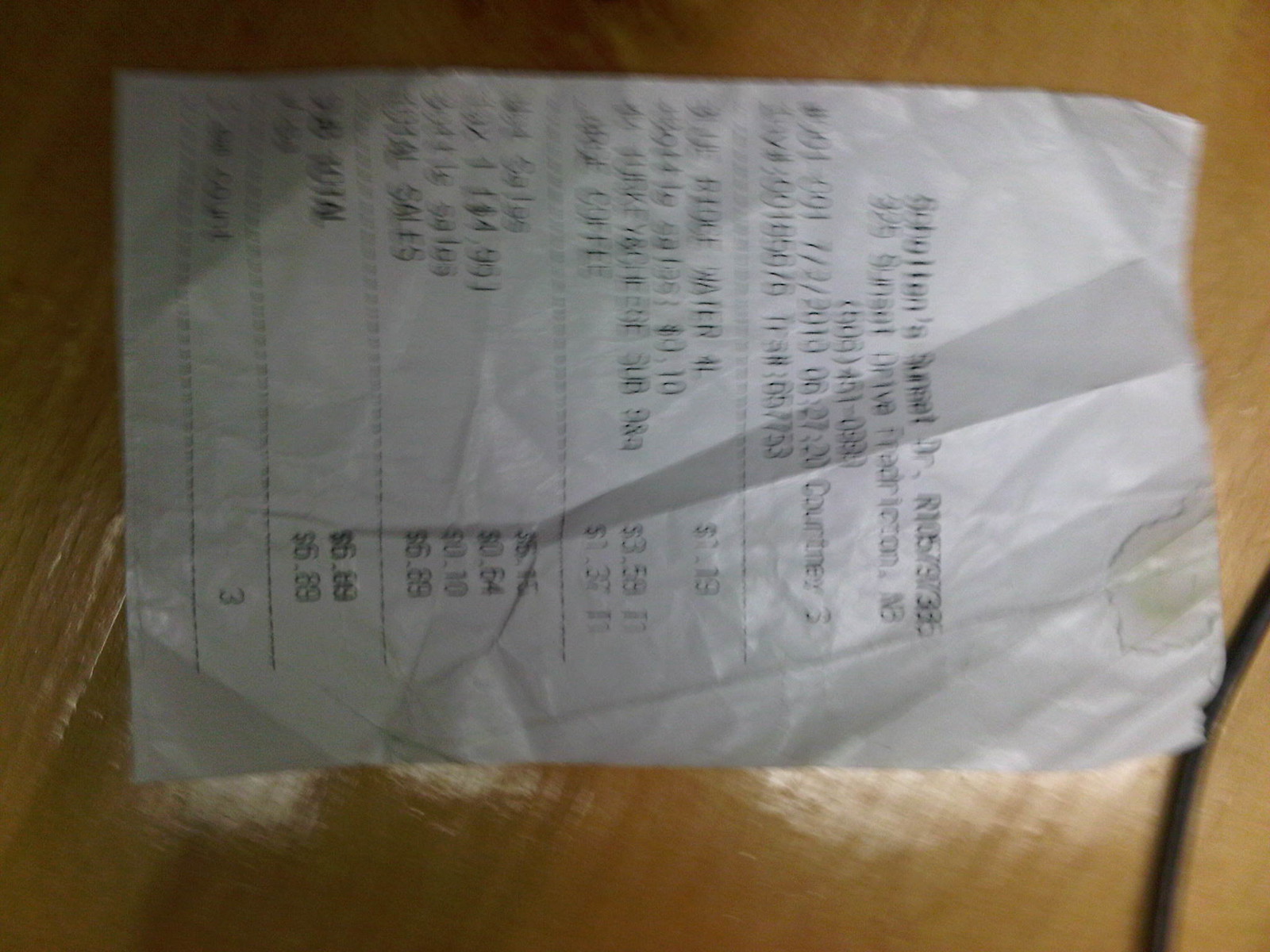This is a blurry photograph of a crumpled and slightly folded white receipt paper lying horizontally on a brown cardboard box. The receipt is twisted sideways, making it difficult to read without tilting your head. Due to the poor image quality, most of the text on the receipt is illegible. However, a noticeable crease runs across the top portion of the paper. Despite the blurriness, the area code visible on the phone number suggests that the business is likely located in the USA.